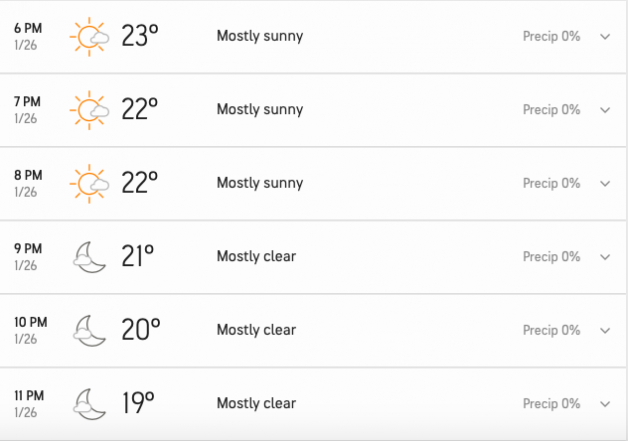Here is a cleaned-up and detailed descriptive caption:

---

The image depicts a detailed weather forecast for January 26th, displayed in a structured format starting from 6 p.m. and ending at 11 p.m. The leftmost column lists the times in hourly increments: 6 p.m., 7 p.m., 8 p.m., 9 p.m., 10 p.m., and 11 p.m. Adjacent to each time slot is an icon representing the weather conditions. At 6 p.m., 7 p.m., and 8 p.m., the icon shows a sun partially obscured by a cloud, indicating partly cloudy conditions. From 9 p.m. to 11 p.m., the icon changes to a moon partially obscured by a cloud, suggesting partly cloudy night skies.

Next to the weather icons, a column specifies the temperature in degrees Fahrenheit, starting with 23°F at 6 p.m. and gradually decreasing to 19°F by 11 p.m. The temperature sequence reads 23°F, 22°F, 22°F, 21°F, 20°F, and 19°F.

Above the weather icons, the third column describes the general forecast conditions: "Mostly Sunny" for each time slot from 6 p.m. to 8 p.m., and "Mostly Clear" for each time slot from 9 p.m. to 11 p.m.

The rightmost side of the image indicates the precipitation percentage, consistently showing 0% for all the listed times. Each box has a downward-pointing arrow at the end, perhaps denoting further details or a continuation of information elsewhere.

---

This structured and detailed caption provides a comprehensive description of the weather forecast image, covering all essential elements clearly.